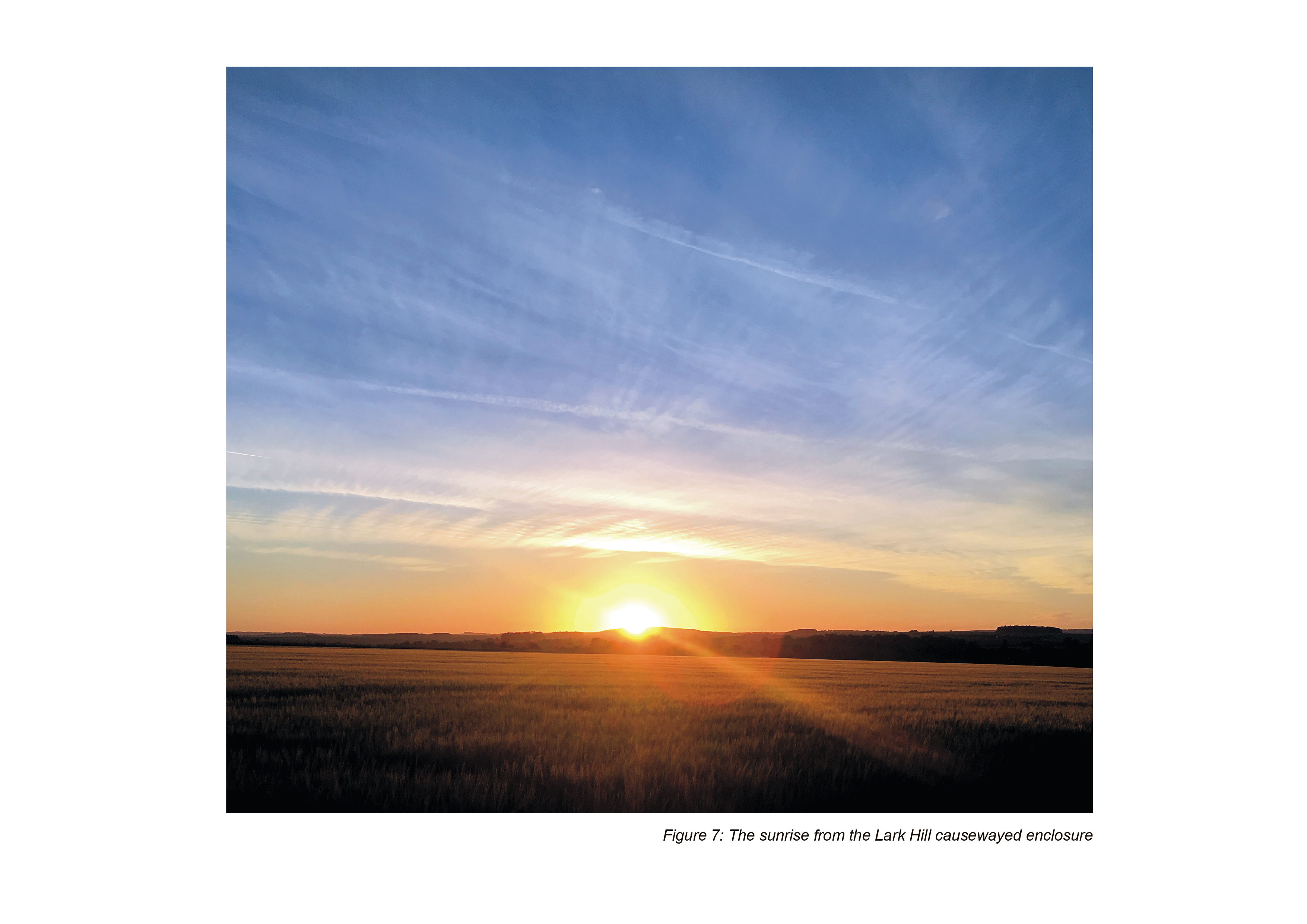This image captures a serene sunrise at Lark Hill Causewayed Enclosure. At the bottom of the photograph, there's a white bar blending into the background with the caption, "Figure 7, the sunrise from Lark Hill, Causewayed Enclosure," written in black, slightly italic text. The sunrise scene features the sun peeking halfway above the horizon, casting bright, flayed orange rays over a vast, flat field covered with wheat or barley. The field extends towards the horizon, which is marked by a line of trees, possibly tumbler trees, and a distant mountain range. The sky transitions from a deep blue at the top to a warm orange near the horizon, adorned with wispy, horizontal clouds. To the right, a building might be faintly visible. The composition is free of any human presence, emphasizing the natural beauty of the landscape.